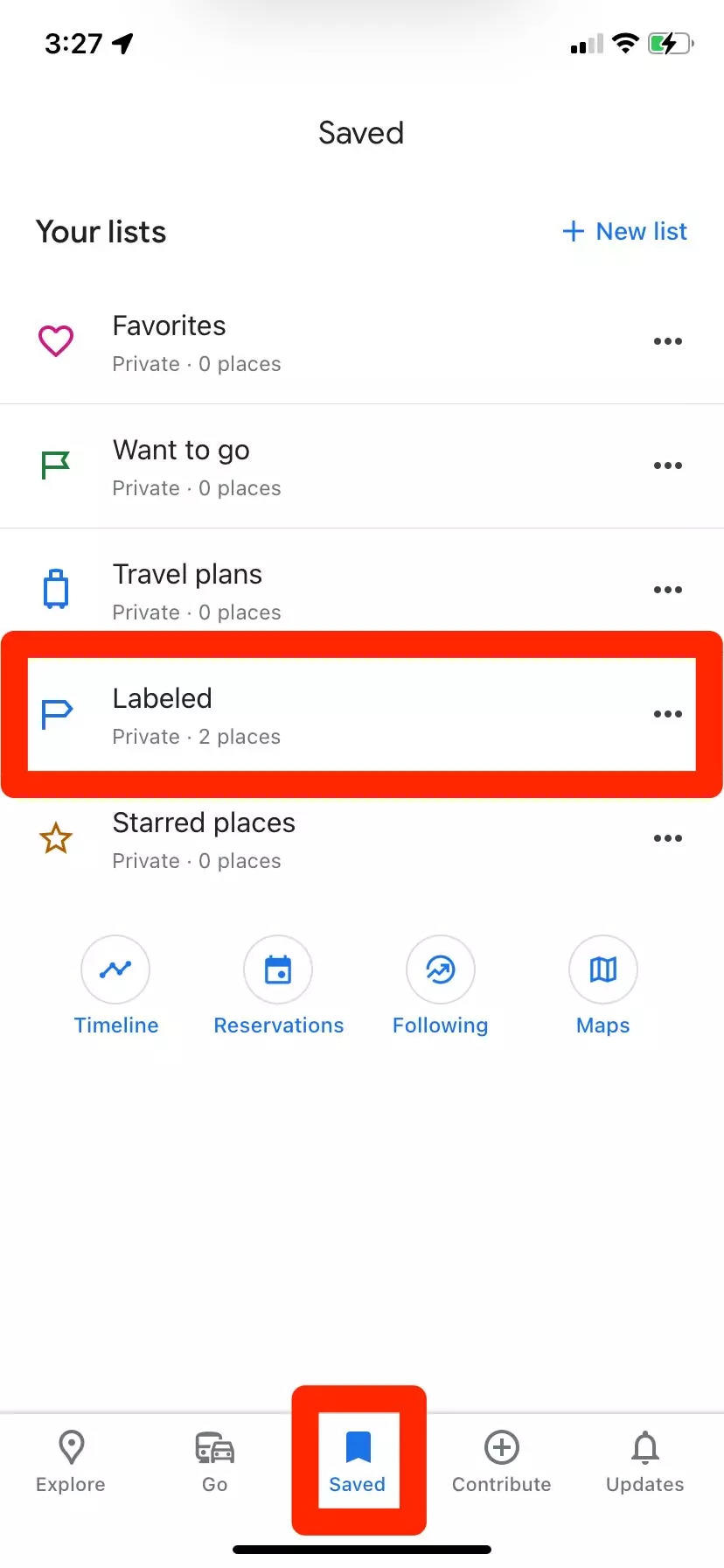A detailed screenshot of a smartphone display showcases various elements of a location-saving application. At the top, the status bar indicates the time as 3:27 PM, depicted with an up-arrow beside it. The internet connection strength shows only two bars, yet it appears stable. The battery icon suggests approximately one-third of the battery life is remaining.

Below the status bar, the main screen of the application features a header labeled "Saved," with an option to add a new list. A series of categorized lists follow this header:

1. A heart logo icon denotes the "Favorites" list, which currently has zero private places.
2. A flag icon next to "Want to go" indicates another private list with zero places.
3. A suitcase icon represents the "Travel plan" list, also with zero private places.
4. A "P" logo for a list titled "Labeled" is highlighted with a red rectangle, indicating a selection or focus. This contains two private places.
5. A gold star logo signifies "Starred places," which presently has no entries.

Additional functional icons reside at the bottom of the screen, representing "Timeline," "Reservations," "Following," and "Maps." The bottom navigation bar highlights options such as "Explore," "Go," and "Save.” The "Save" icon is currently selected, indicated by a red square around it. Further options include a plus button for contributing new locations and an updates tab marked by a bell icon.

This comprehensive snapshot vividly captures the app's categorized lists and functional navigation, detailing the smartphone's status indicators and user interface elements.